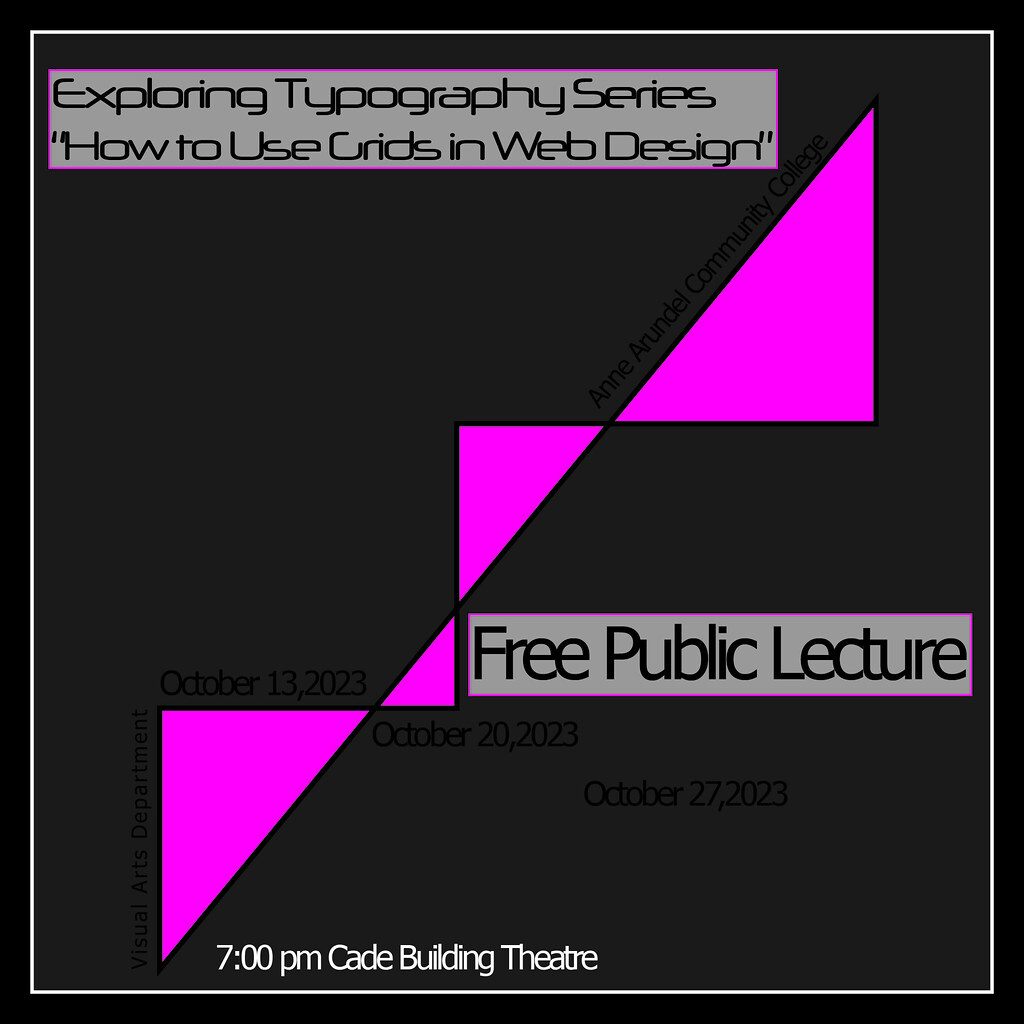The image is a digitally designed advertisement, likely created using software such as Photoshop, with a dark gray border and a white inner border set against a brown background. At the top left, a light gray box with a hot pink border contains the text "Exploring Typography Series: How to Use Grids in Web Design" in dark gray font. Diagonally across the image, there are four obtuse triangles of varying shapes and sizes, all in pink. The largest triangle at the bottom points up and contains the text "Visual Arts Department, October 13, 2023" in black, while a smaller triangle next to it points down and says "October 20, 2023". Other important details include the location and time of the event, noted at the bottom of the advertisement as "7 p.m. Cade Building Theater." The ad also mentions "Anne Arundel Community College" in black text, indicating the hosting institution. This visually striking advertisement combines a variety of text elements and geometric shapes to promote a free public lecture series on typography and web design.